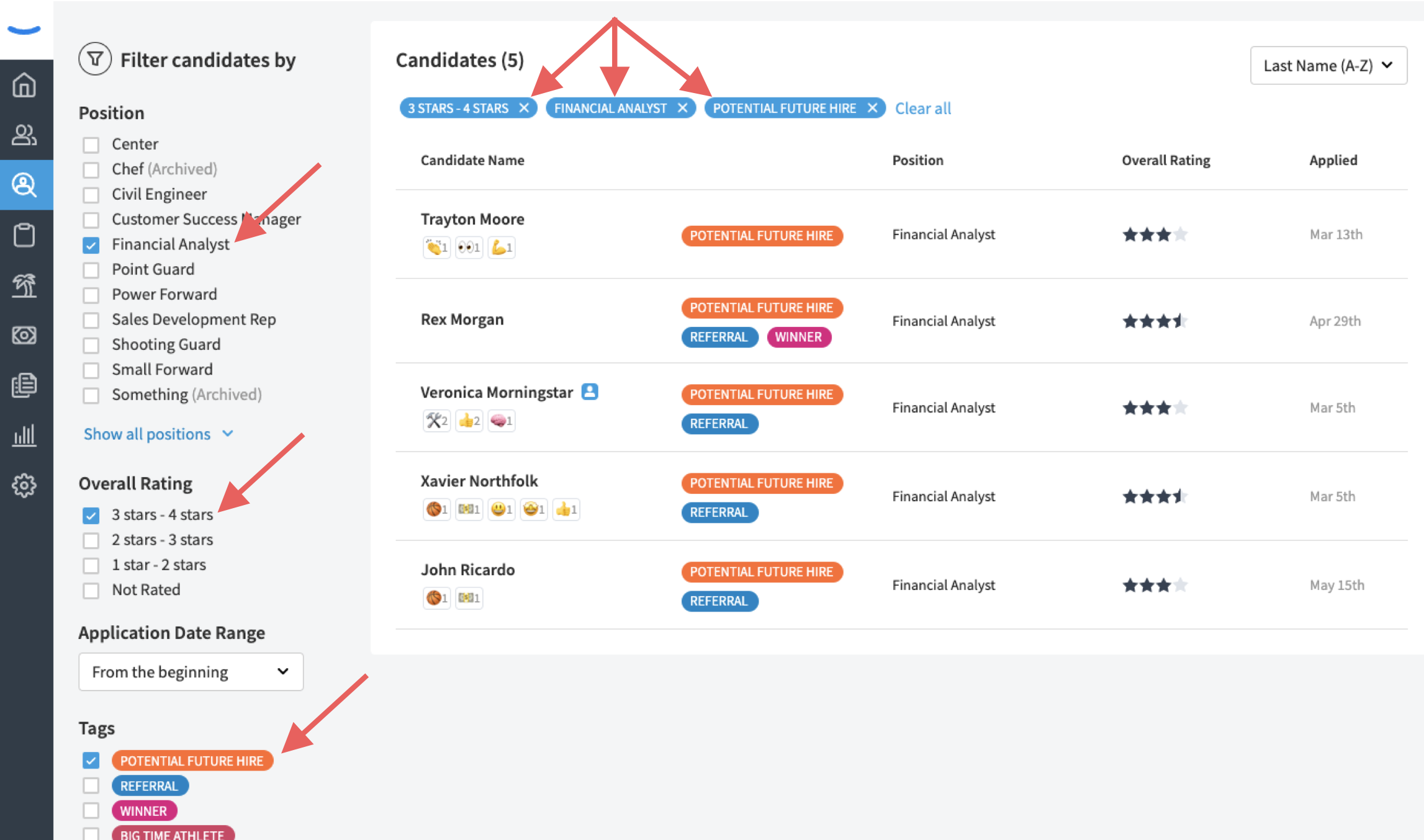The image shows a screenshot from a computer displaying a candidate filtering and rating interface. On the far left, there is a vertical black column with various icons, in order from top to bottom: a house, two people, a magnifying glass with a person inside, a square, a palm tree, a dollar bill, a document, a bar graph, and a settings gear.

Next to this column is a larger gray box titled "Filter Candidates by Position". Below this title, there are multiple selectable categories for filtering. The section includes an "Overall Rating" filter with options to check various rating levels, and an "Application Date Range" filter option.

Highlighted within the screenshot are specific candidates and filters. Arrows point to the "Financial Analyst" category, indicating filters set to show candidates rated between three and four stars, and an area labeled "Potential Future".

A pop-up rectangle on the screen titled "Candidates (5)" displays a list of five candidates:
1. Treyton Moore
2. Rex Morgan
3. Veronica Morningstar
4. Xavier Northfolk
5. John Ricardo

Below each candidate's name is detailed chart information, presumably outlining their qualifications and fit for the position.